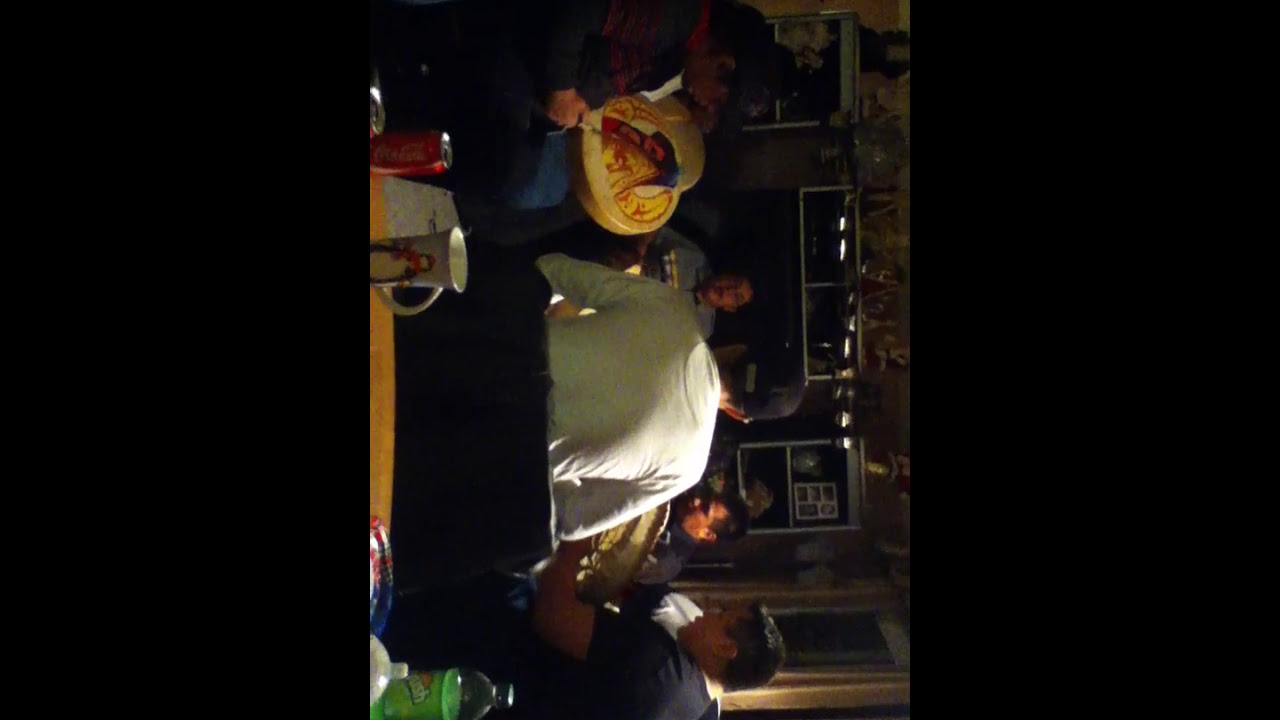This is a sideways image, oriented 90 degrees clockwise, depicting a dimly lit, indoor scene. Several men, all with dark hair and some wearing hats, are seated around a table. The man at the center has his back to the camera, obscuring much of the table's surface and creating difficulty in discerning what they are doing. They appear to be engaged in an activity that involves holding and possibly carving or assembling objects, rather than eating. 

In the foreground, there is a table with some items: a green bottle of Crush soda, a Coca-Cola can, a cup with a penguin illustration, and several plates and cups. Behind the men, there are shelves with various objects and what seem to be air conditioners or air ventilators, suggesting an indoor home or restaurant setting. A window with a curtain on the right side lets in some light, adding to the overall dim ambiance of the room.